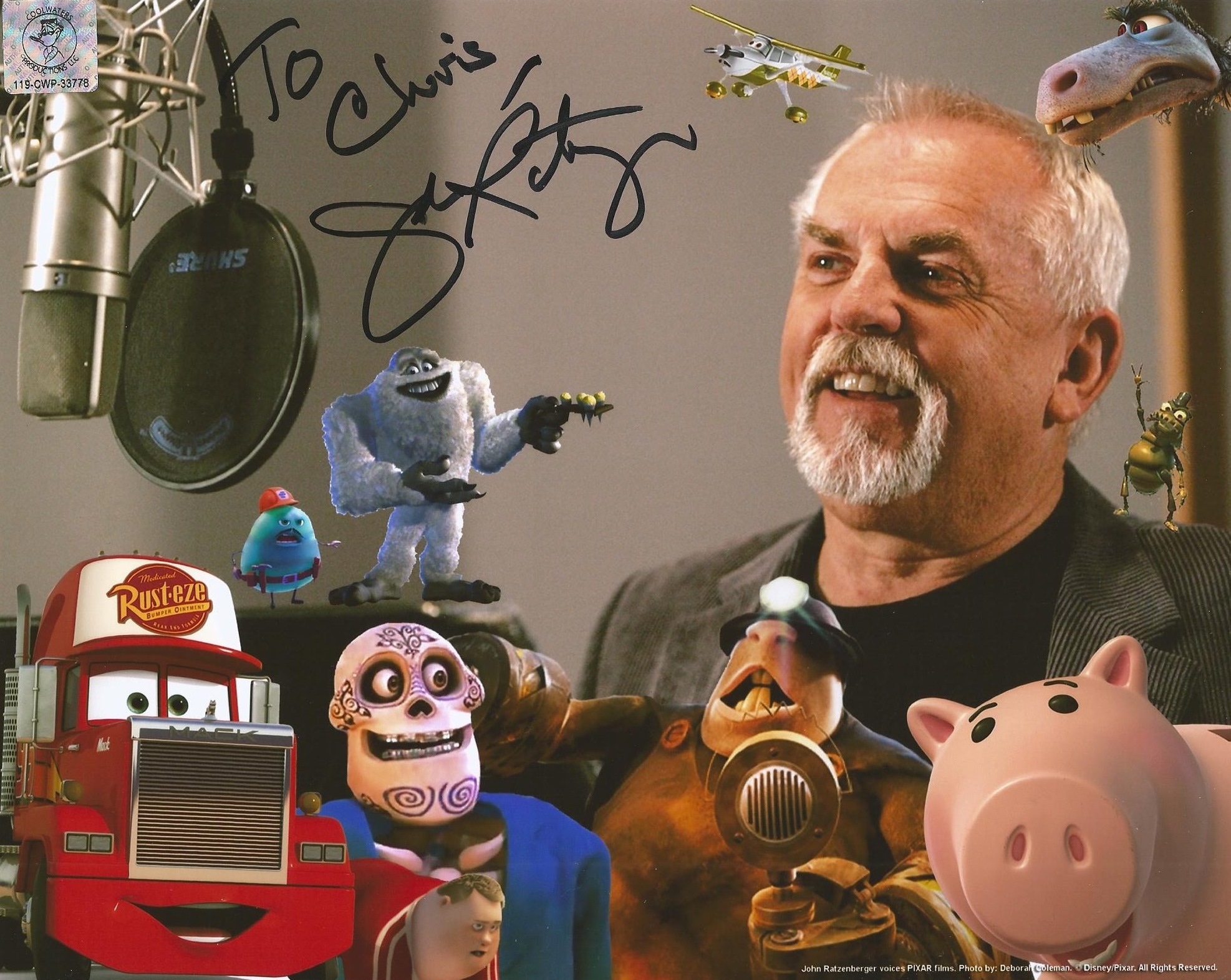The image depicts an indoor setting, likely a radio station, featuring a man centered in the frame and smiling, with short grey and white hair and a white goatee. He is dressed in a grey-and-black pinstriped jacket over a black t-shirt. In the top left corner, a microphone hangs down near an autograph that reads "To Chris," alongside the man's signed name. A small, out-of-focus symbol featuring a character can be seen in the upper right corner. The background is grey, and lining the bottom of the image are various toys, including Rusty the Mack truck, characters from Monsters, Inc., and a piggy bank likely from Toy Story. Additional toys include an airplane from the Cars movie and a skeleton character in a suit. The colors visible in the image include light brown, black, grey, blue, purple, tan, pink, red, orange, yellow, and light blue. This photo appears to be an autographed picture.